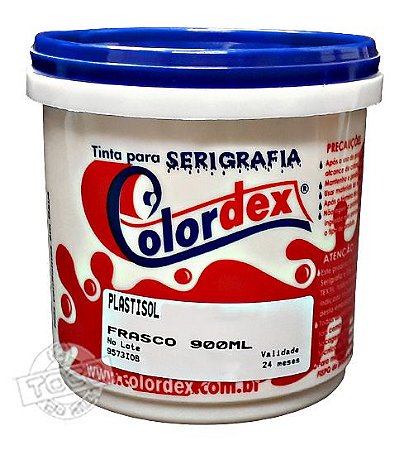This image features a close-up of a container prominently branded as "Color Dex". The container, which appears to be a 900-milliliter jar, has a vibrant design: the upper portion is white and the lower half sports a dynamic, wavy red pattern. The word "Color Dex" stands out, with "Color" in blue and "Dex" in red, underlined with a blue ribbon originating from the 'C'. A royal blue lid tops the container.

A white label with black text covers a significant part of the container's front, reading "frasco 900 milliliters" and "Plastisol," suggesting that it's likely some kind of plastisol-based product, possibly used in screen printing, given the "tinta para serigrafia" text which translates from Spanish to "ink for screen printing". A transparent logo near the bottom left reads "TOC". The container also features a web address, "colordex.com.br", indicating a Brazilian origin. The background of the image is plain white, further highlighting the detailed branding and design of the container.